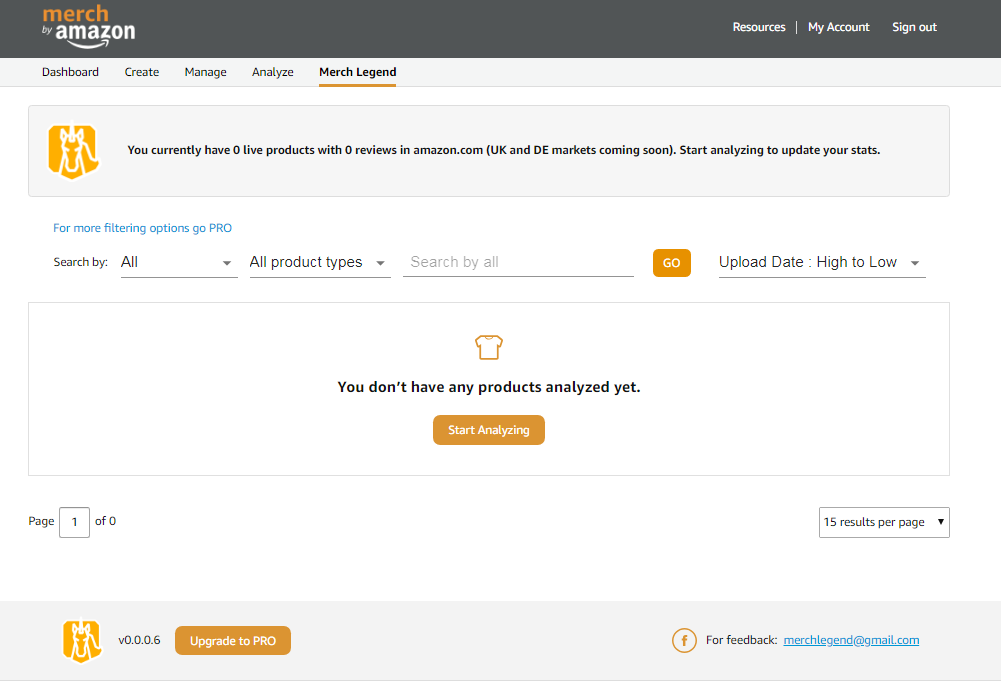**Descriptive Caption:**

The image depicts an Amazon Merch dashboard interface. At the top left corner, "Merch by Amazon" is prominently displayed on a slate gray strip. On the right side of the strip, there are options for "Resources," "My Account," and "Sign Out." 

Beneath the top strip, a navigation panel can be seen on the left, listing: Dashboard, Create, Manage, Analyze, and Merch Legend, with an orange line underlining "Merch Legend." Below this, a unicorn head icon sits within a shield-like shape, facing forward. The message "You currently have zero live products with zero reviews in amazon.com (UK and DE markets coming soon). Start analyzing to update your stats," appears against a gray background, differentiating from the mostly white page. 

Further down, there is a blue link stating "For more filtering options GoPro," followed by a search bar with drop-down options for filtering by "All products/types" and an orange "Go" button. Adjacent to the search bar is another drop-down labeled "Upload Date: High to Low."

An outlined rectangle, positioned below, contains a t-shirt icon and the message "You don't have any products analyzed yet." Accompanied by an orange "Start Analyzing" button with white text, inviting users to interact.